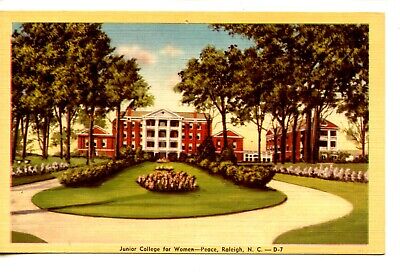This postcard features a picturesque drawing of the Junior College for Women in Peace, Raleigh, North Carolina, identified by the black text at the bottom reading "Junior College for Women, Peace, Raleigh, N.C. D7." The main building, with its distinctive red brick facade and white gabled front, stands prominently in the background. This central structure is accented by a gabled white porch and a matching red gabled roof. Flanking this building are smaller red brick buildings, also adorned with white roofs.

A long plot of green grass, dotted with colorful flowers and shrubbery, stretches out before the building, split by a central walkway. The pathway is bordered by additional rows of flowers and bushes. Tall trees with green leaves and white flowers at their base frame the scene on both the left and right sides. The sky overhead is a soft blue with scattered white clouds, adding to the serene outdoor setting. Surrounding the image is a light yellow border, enhancing the vintage charm of this old-fashioned postcard.